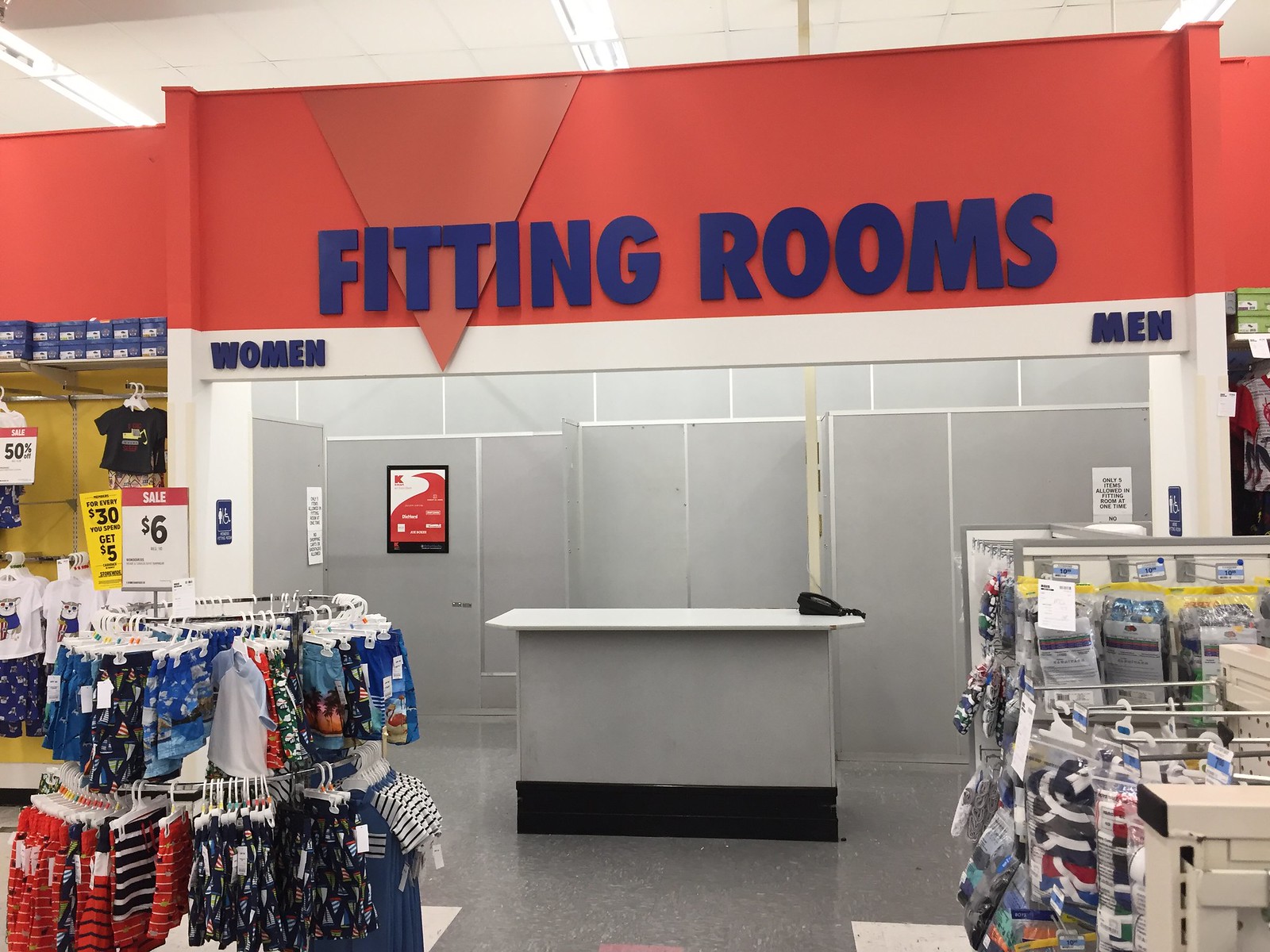The image depicts a fitting room area within a Kmart department store, identifiable by the prominent red banner with "Fitting Rooms" inscribed in large blue letters and the characteristic Kmart "K" logo. The fitting rooms are clearly divided, with the women's section on the left and the men's section on the right, each featuring a handicapped stall. A table, likely for an attendant, sits in front of the fitting rooms, possibly with a telephone placed on it. To the left, there is a display of children's swimwear on sale for $6. On the right, racks hold items encased in plastic bags, including boxer briefs for kids. The area is marked by a clean, grayish-white floor. Additionally, signs on the doors indicate restrictions such as a five-item limit in the fitting rooms at one time. The walls feature additional clothing and shoe storage, characterized by shoes in boxes and shelves with socks or underwear. The entire scene conveys an organized yet bustling retail environment.